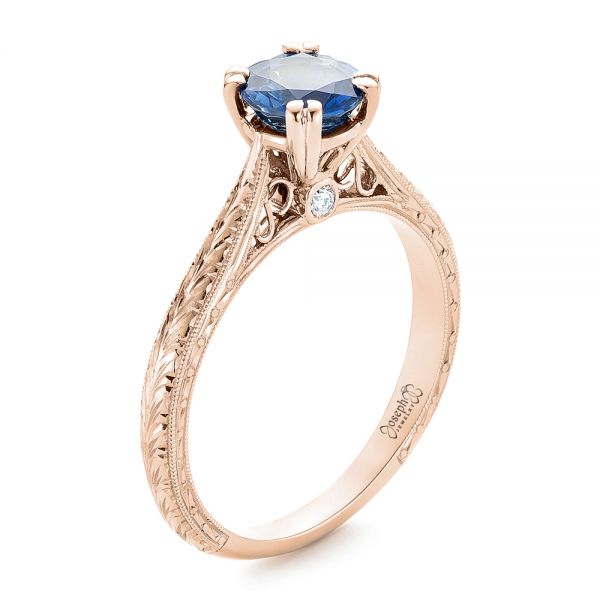This close-up product photograph showcases an ornate and intricately designed ring, primarily presented against a stark white background with minimal shadowing. The ring features a pale, subtle gold hue with a slight pinkish tint, creating a refined and elegant look. The band is adorned with elaborate scrollwork and leaf-like patterns, enhancing its overall decorative appeal. Along the edges, a dotted ridge accentuates the intricate craftsmanship. 

At the center of the ring, four small golden prongs securely hold a faceted, royal blue gemstone, possibly a sapphire, which is both reflective and eye-catching. Just beneath this prominent blue gem, a smaller, clear, faceted stone, which might be a diamond, is set into the band, visible only from a certain angle.

Inside the ring, the inscription reads "Joseph Jewelry" in black, accompanied by a stylized logo that resembles a butterfly or a series of overlaid 'J' letters. The ring’s rich design and fine details underline its luxurious and unique character, making it a standout piece of jewelry.